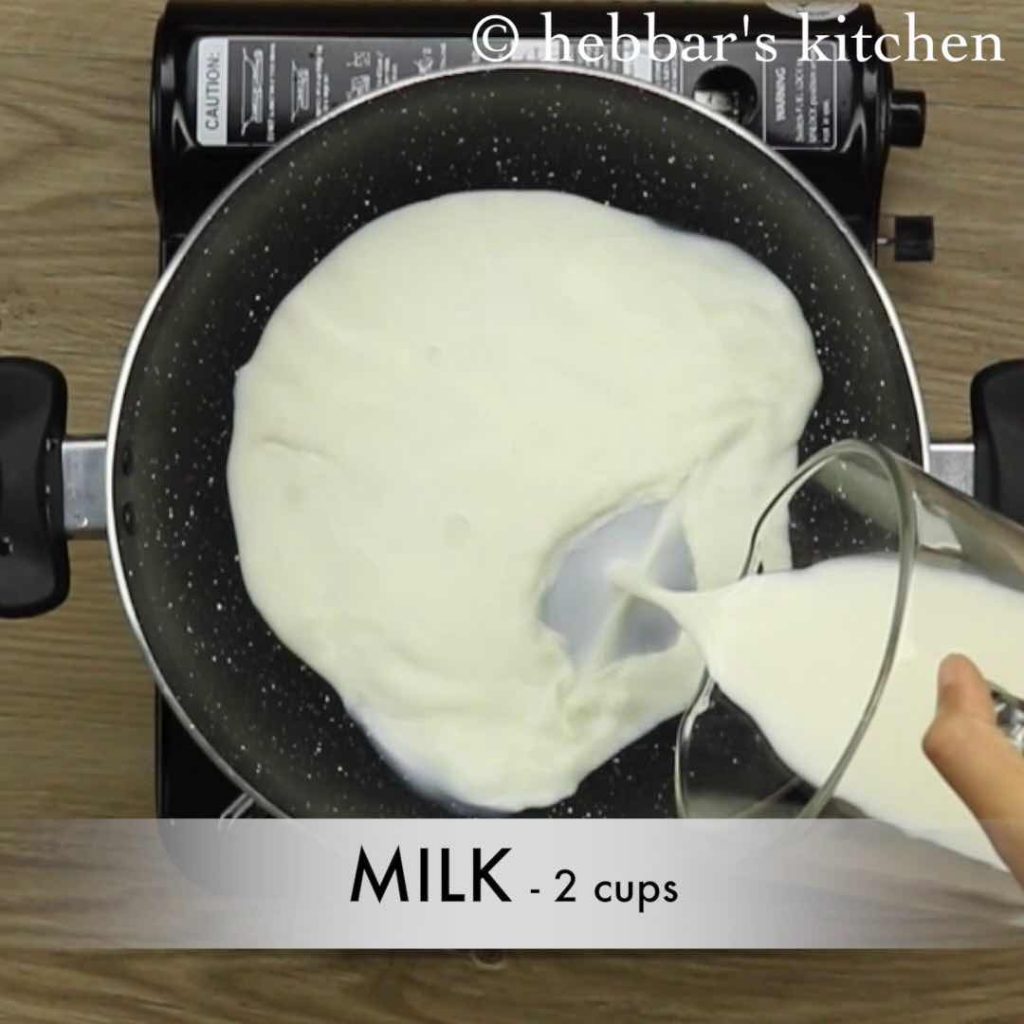The image is a still from a video, likely a cooking show or recipe tutorial from Hebbar's Kitchen (copyright "H-E-B-B-A-R apostrophe S, KITCHEN" in white font at the top right corner). The shot, taken from a top-down angle, features an induction cooker placed on a light-to-dark brown wooden surface. Centered in the frame is a large, gray non-stick frying pan with white specks, equipped with two side handles (thin metal rods with black ends visible on both sides of the pan). 

At the bottom right, a hand is seen pouring milk from a large glass jug into the pan, with the thumb gripping the top handle of the jug. Underneath this scene, a semi-transparent, soft white banner displays the text "MILK, 2 CUPS" in large black, capital letters. The pan also displays a small propane tank or an "induction base caution sticker" above it, adding a sense of depth and safety awareness to the image.